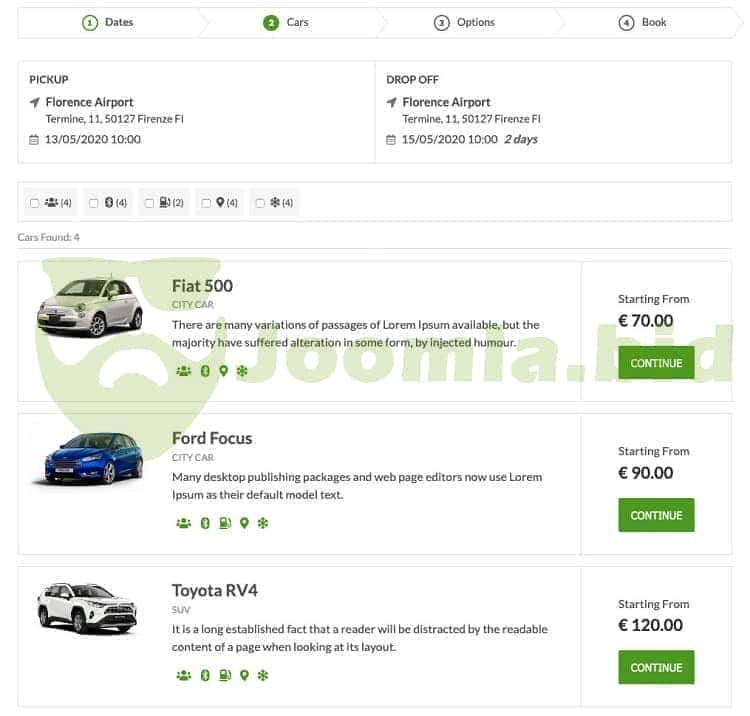The screenshot depicts the user interface of Joomla.bid, which appears to be a car rental platform. 

**Upper Section:**
- At the top-left corner, there are navigation buttons labeled: "Dates," "Cars," "Options," and "Book," organized in a sequence. Currently, the "Cars" section is active, indicated by a green circle with the number two inside it.

**Details Section:**
- Below this navigation bar, there are two rectangular boxes labeled "Pickup" and "Drop Off."
    - **Pickup:** 
      - Location: Florence Airport
      - Date and Time: Specified for a two-day rental period
  - **Drop Off:**
      - Location: Florence Airport (same as pickup)
      - Date and Time: Corresponding with the pickup details, indicating rental duration

**Filters Section:**
- Directly beneath the location/date-time details, there is a smaller rectangular bar providing options to filter cars based on features like Bluetooth, fuel type (gas), etc.

**Cars Selection:**
- The interface displays a selection of cars in three rectangular sections, each representing a different car model. Above these sections is a header indicating the total number of cars found ("Cars Found: 3").
  - **First Car:**
    - **Model:** Fiat
    - **Price:** 70 Euros per day
    - **Action:** Green "Continue" button
  - **Second Car:**
    - **Model:** Ford Focus
    - **Price:** Starting at 90 Euros per day
    - **Action:** Green "Continue" button
  - **Third Car:**
    - **Model:** Toyota RAV4
    - **Price:** Starting at 120 Euros per day
    - **Action:** Green "Continue" button

Each car listing includes its name and a brief description, accompanied by a price column and a corresponding "Continue" button, facilitating further steps in the booking process.